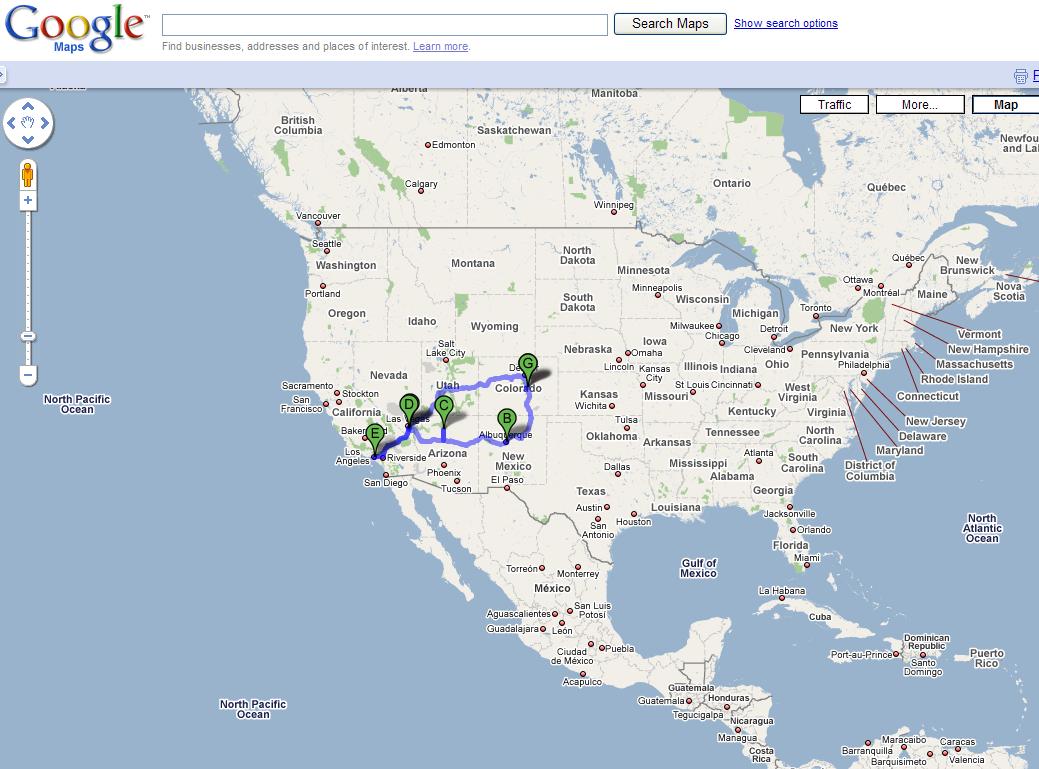This image is a screenshot from Google Maps displaying a detailed map of the United States and parts of Canada, Mexico, and the surrounding oceans. At the top, the Google logo and Google Maps branding are visible, along with a search field, a "Search Maps" button, and a hyperlink for "Show Search Options."

The map features a light blue ocean background: the North Pacific Ocean is to the left, the Gulf of Mexico is central, and the North Atlantic Ocean is to the right. The map highlights the entire United States, Canada from British Columbia to Newfoundland, and a portion of Mexico and South America.

Five specific locations within the U.S. are marked with green, upside-down teardrop-shaped pins containing black capital letters. These pins signify a suggested driving route through:

- Point B: Albuquerque, New Mexico
- Point C: Northern Arizona
- Point D: Las Vegas, Nevada
- Point E: Los Angeles, California
- Point G: Denver, Colorado

The route is illustrated with a connecting blue line through these points, depicting a loop that starts and ends at Albuquerque, showing directionality in the specified travel path. Additional map elements include black labels for U.S. states and countries, and a navigational zoom bar on the left side of the image.